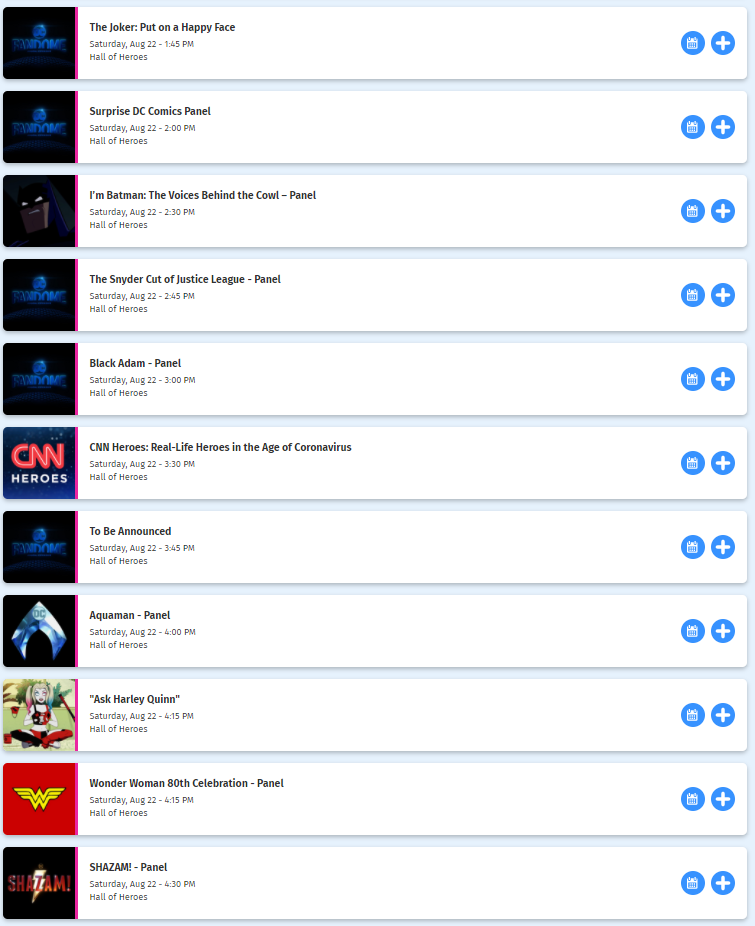This is a detailed screenshot of an event listing, seemingly for a convention focused on DC Comics. Each event is organized in rows and stacked vertically, resembling a schedule format, perhaps for a day-long or multi-day convention.

At the top of the list is an event titled "The Joker: Put on a Happy Face", scheduled for Saturday, August 22 at 1:45 PM, located at the Hall of Heroes. Adjacent to each event listing are icons for adding the event to a calendar and a plus button for additional actions.

Following the Joker event, there is a "Surprise DC Comics Panel", hinting at a potentially special or unexpected presentation. Subsequent listings include:

- "I'm Batman: The Voice Behind the Cowl Panel"
- "The Snyder Cut of Justice League Panel"
- "Black Adam Panel"
- "CNN Heroes: Real Life Heroes in the Age of Coronavirus"
- "To Be Announced (TBA)"
- "Aquaman Panel"
- "Ask Harley Quinn" session
- "Wonder Woman 80th Celebration Panel"
- "Shazam Panel"

The layout and content suggest this is a comprehensive schedule of panels and discussions, offering attendees information about various events they can attend, complete with dates and times.